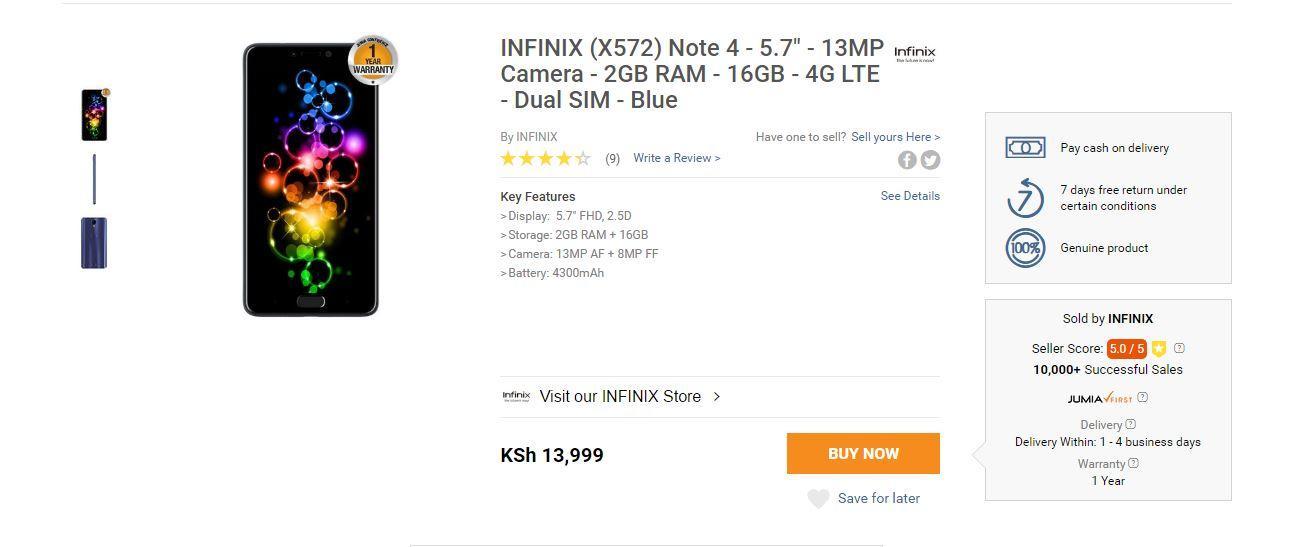![Infinix Note 4 Smartphone Available on Online Store]

This image showcases an Infinix Note 4 (X572) smartphone listed on an online store. The phone is prominently displayed on the left side with a circular badge at the top, possibly indicating a top-selling item. 

The listed specifications include:
- Model: Infinix X572 Note 4
- Display: 5.7-inch FHD
- Camera: 13 MP 
- RAM: 2 GB
- Storage: 16 GB
- Connectivity: 4G LTE
- Features: Dual Sim
- Color: Blue
- Battery: 4300 mAh

The phone has received a 4-star rating and is marketed by Infinix. The price is listed as KSH 13,199. Customers are given the option to purchase immediately or save the item for later. 

Seller and purchase details are provided:
- Payment Options: Cash on delivery
- Seller: Genuine products sold by Infinix; seller's score 5875 with over 10,000 successful sales
- Delivery: Jumai delivery within one to four business days
- Warranty: One year warranty
- Additional Offer: "Have one to sell? Sell yours here."

The description also highlights some customer-friendly policies, including a 7-day free return under certain conditions and a free forum for user discussions.

**Visit the Infinix Store** on the platform to explore more products and deals.